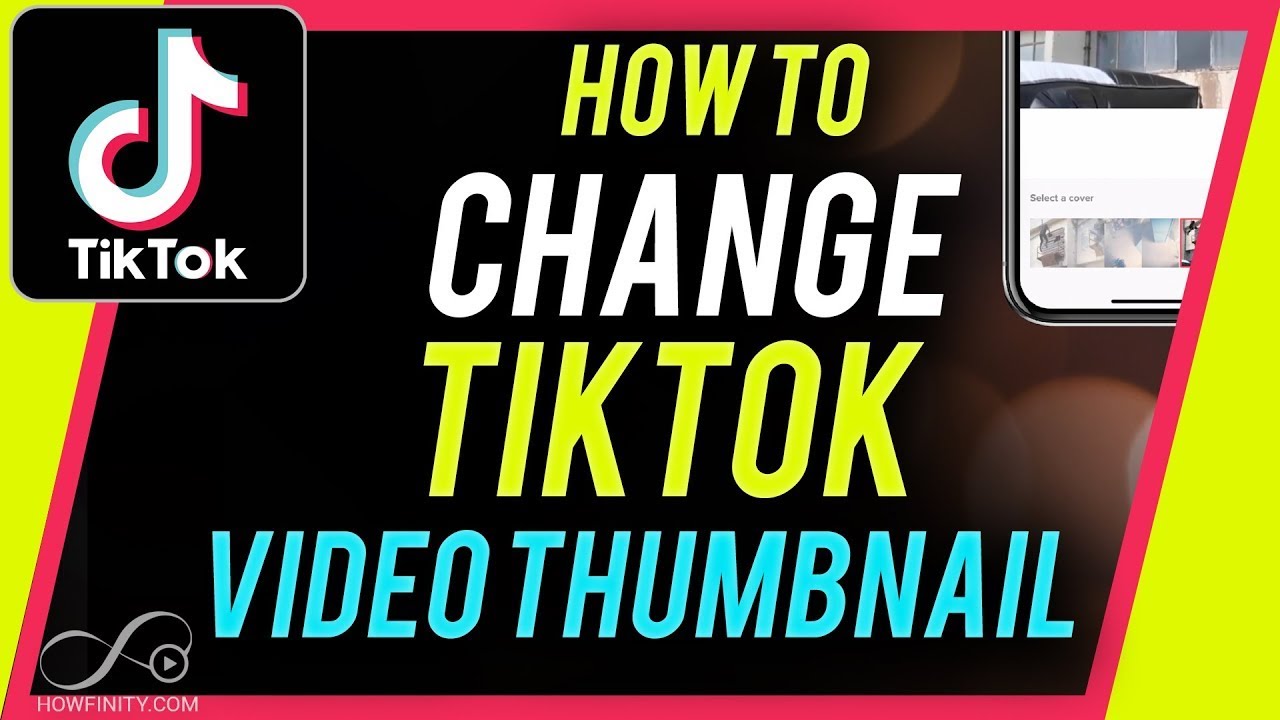The image is a colorful and detailed rectangular graphic. Both the very left and right sides are filled with a vibrant neon green color. In the center, there is a prominent red-bordered parallelogram serving as a focal point. The left background within the parallelogram is black, while the right background is a brownish shade with light circular glares.

In the upper left corner of the image, a black square with a white border features the iconic TikTok symbol in white, blue, and red. Below this, the word "TikTok" is written in white.

Across the parallelogram, various texts appear in different colors. The top line, in neon green, reads "How to." Below this, in a larger white font, the word "Change" is displayed. Beneath it, the word "TikTok" is again in neon green, followed by "Video Thumbnail" in light blue.

In the lower left corner, a white infinity symbol, resembling a sideways number eight, is present next to the text "howfinity.com," also in white.

The upper right corner of the image reveals the edge of a phone screen. Zooming in, the screen displays the text "Select Cover" in black. The screen shows what appears to be a series of images or windows, with the first image depicting a person standing near a window, although the details are somewhat indistinct.